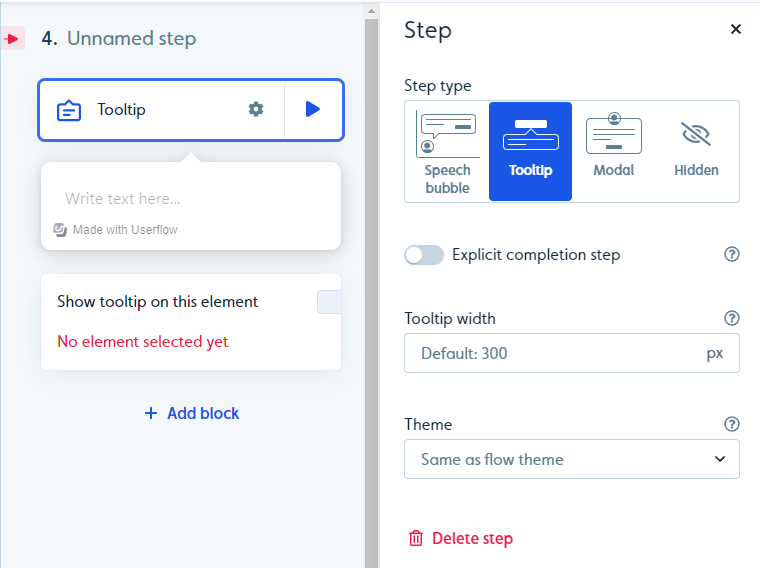The image depicts a user engaging with a UI design application. The screen is divided into two sections displayed side-by-side. On the left side, there is an element labeled as 'Unnamed Step' accompanied by the placeholder text 'Write text here.' Below this, a button labeled 'Show Tooltip on this Element' is visible. When clicked, it opens various customization options for the tooltip. These options include setting the tooltip width, which has a default of 300 pixels, and selecting the tooltip's theme, which matches the overall flow theme by default. The detailed elements and configurable settings suggest that the user is in the process of designing a user interface, tailoring specific elements such as tooltips and speech bubbles, each with their own customizable properties and methods, indicating a technical and highly customizable design environment.